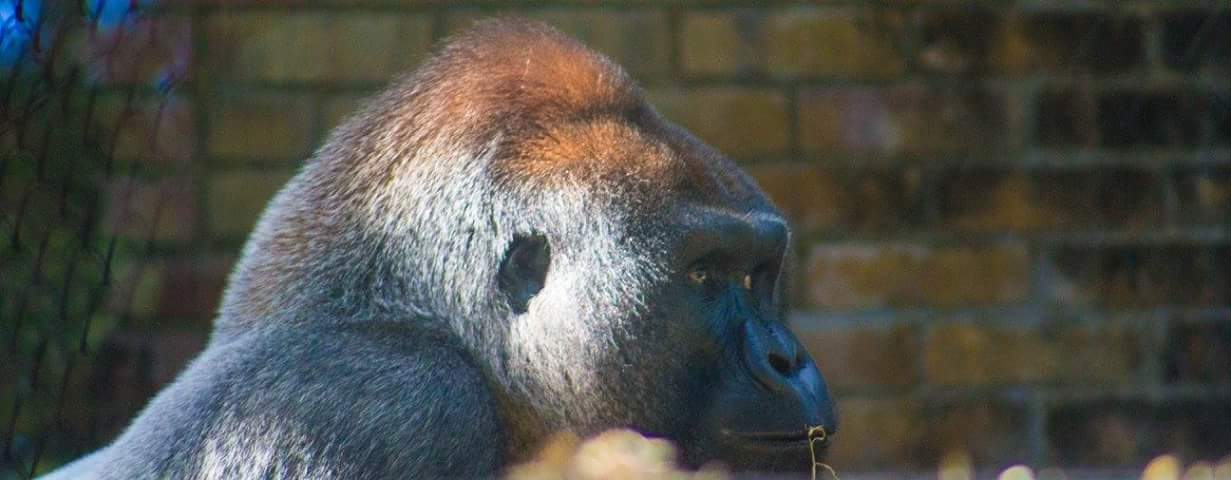The photograph captures the upper body of a silverback gorilla, from the shoulders up, with the gorilla facing towards the right in a side-view portrait. The top of the gorilla's head features bright, orange-brown hair, while the rest of its fur is predominantly black. There appears to be a silver or gray tint to the hair on the side of its head, possibly due to lighting. The gorilla's eyes are a striking yellow or green. A piece of grass protrudes from its mouth, adding a dynamic element to the image. In the background, there is a weathered brick wall that is primarily yellow with some red sections on the right side. Additionally, a chain-link fence is visible, with light from an adjacent structure filtering through it, suggesting the setting might be a zoo, indicating the gorilla is in captivity.